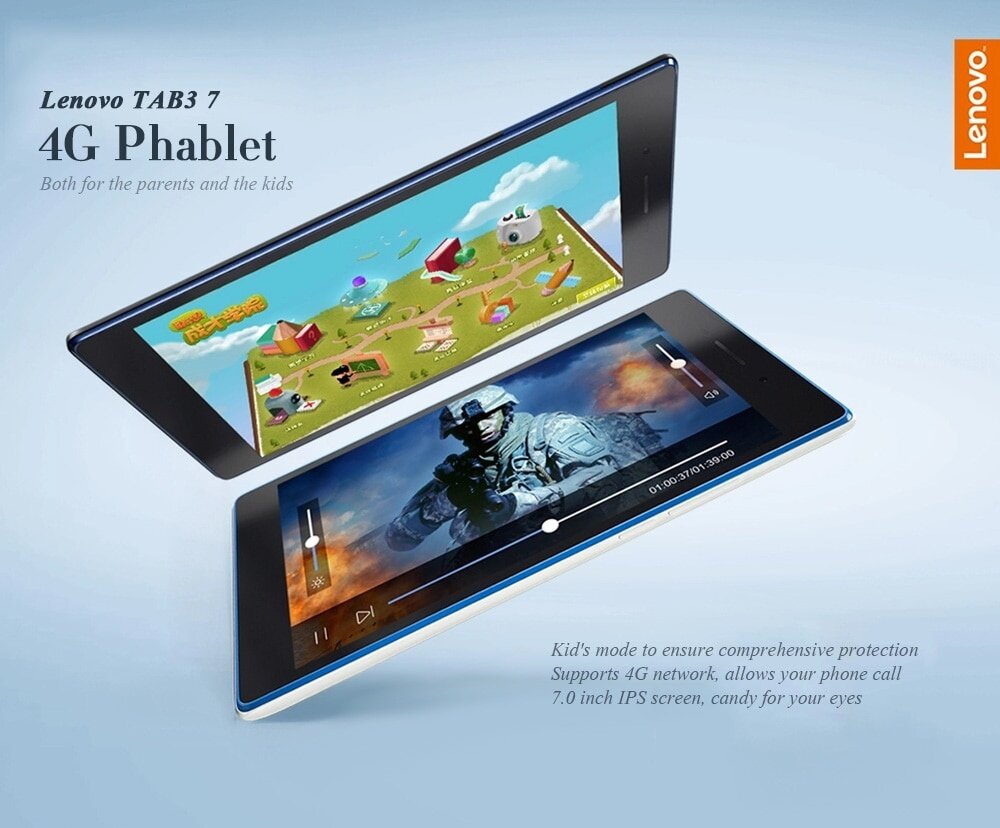This full-color square image is an advertisement for the Lenovo Tab 3 7 4G Phablet. The background is primarily blue, with the notable presence of logos. At the upper right corner is the red Lenovo logo with white text. Meanwhile, the upper left corner features a black logo for the Lenovo Tab 3 7 4G Phablet. The same logo also appears in the lower right hand corner. The image showcases two Lenovo Tab 3 7 4G Phablets positioned diagonally to each other, accentuating their features. The tablets are not connected like a laptop but are shown separately displaying different screens. One screen shows a child-friendly interface with bright colors and playful images, possibly in a different language such as Chinese, indicating a kids mode. The other screen displays a more mature scene, possibly from a movie, with a soldier holding a gun. Text on the lower portion of the image highlights key features: "Kids mode to ensure comprehensive protection, supports 4G network, allows your phone call, 7.0-inch IPS screen, candy for your eyes." The tagline underscores the device's appeal for both parents and children.